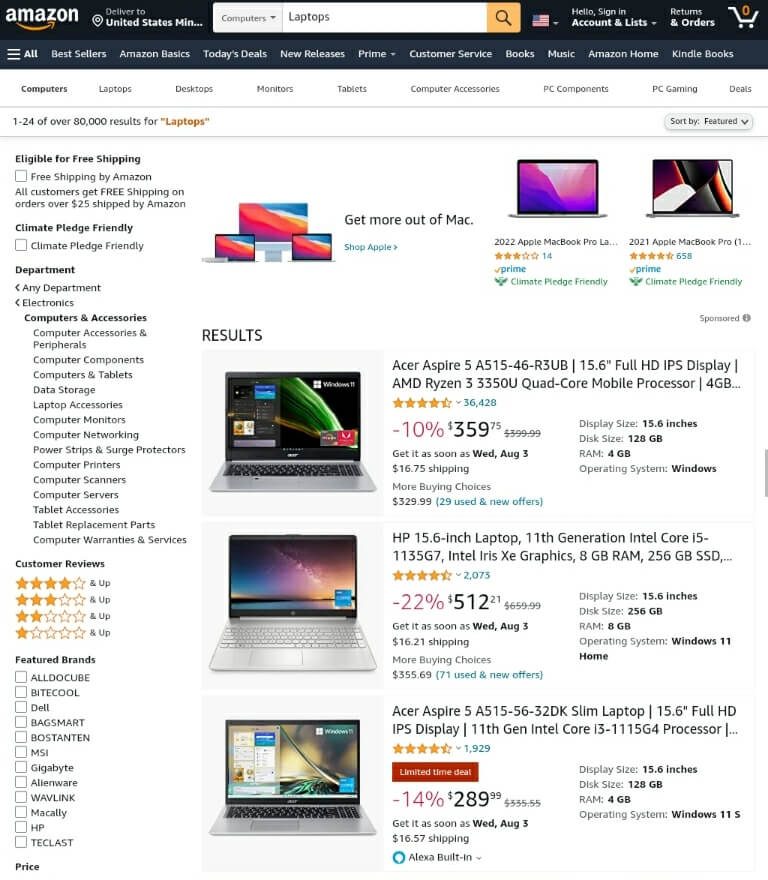A detailed description of the image:

This image showcases an Amazon shopping page focused on laptops. The top portion of the page prominently features the Amazon logo and standard navigational elements, which include links to "Best Sellers," "Amazon Basics," "Today's Deals," "New Releases," "Prime," "Customer Service," "Books," "Music," "Amazon Home," and "Kindle Books." Notably, the user is not signed in, so no personal account information is displayed.

Directly beneath this, a search bar specifically configured for the computers category is visible. The categories listed here include "Computers," "Laptops," "Desktops," "Monitors," "Tablets," "Computer Accessories," "PC Components," "PC Gaming," and "Deals." 

The main content area begins with a section dedicated to various computer accessories and departments, featuring options for "Any Department," "Electronics," "Climbing," "Pledge Friendly," and "Eligible for Free Shipping." Following this, a subsection highlights MacBooks.

The search results for laptops are then displayed, starting with an Acer laptop priced at $359, equipped with a quad-core mobile processor. Below it, an HP laptop with a 15.6-inch display is listed for $512. The most affordable option shown is another Acer laptop, also with a 15.6-inch display, priced at $289. All the laptops mentioned have 15.6-inch displays but vary in processing power and price.

Additionally, there is a feature for filtering results by brand, allowing users to customize their search to include or exclude specific brands. The image captures a comprehensive view of the page, emphasizing the variety and options available for laptop shoppers on Amazon.